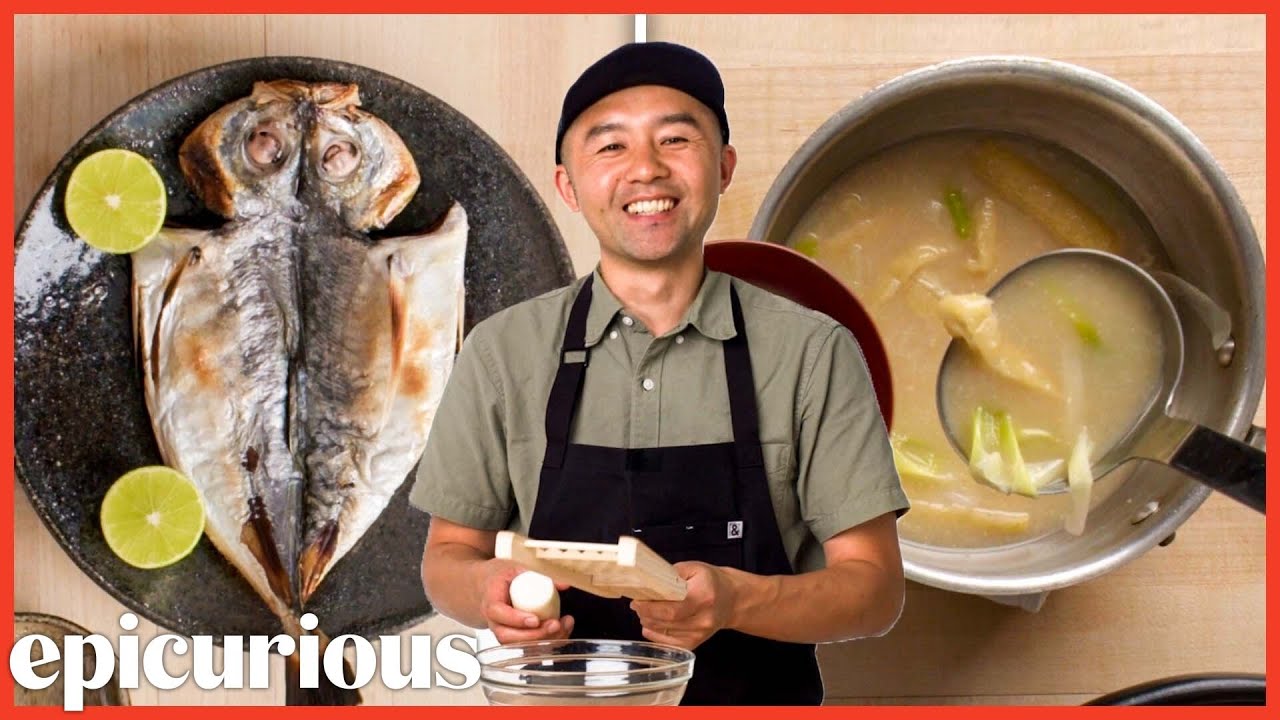The image features an Asian chef prominently positioned in the center, smiling directly at the camera. He wears a green button-up shirt, a black apron, and a small black hat. With his left hand, he holds a cutting instrument and a half daikon radish over a clear round bowl. The background displays two culinary images: on the left is a round black dish containing two skillet-fried fish, accompanied by two half limes; on the right is a creamy-colored soup with green vegetables, being scooped by a large stainless steel ladle with a black handle. The bottom left of the image displays the word "Epicurious."